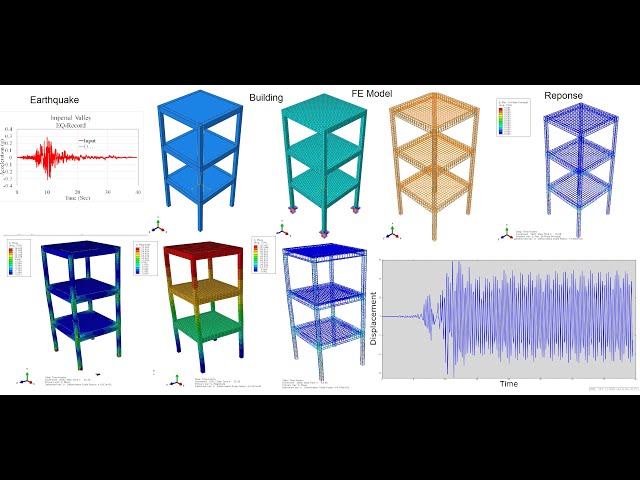The infographic presents a detailed schematic representation of the effects of an earthquake on various buildings, seen through a collection of diagrams and accompanying waveform charts, all set against a white background with a black bar at the top and bottom. At the top left, a red line graph labeled "Earthquake" plots the Imperial Valley EQ record, indicating the force of the earthquake over time. To the right of this graph are four color-coded diagrams of multi-tiered shelf-like structures, each with three tiers and four legs, resembling buildings. These are colored blue, teal, light orange, and dark blue with varying transparencies and configurations. The structures are labeled alternatively as "Building," "FE Model," and "Response," showing different phases or models of analysis. Below these, a second row of diagrams continues with similarly styled structures viewed from a more head-on perspective, featuring color variations including blue with green streaks, a multicolored structure with red, yellow, and green tiers, and another blue wireframe. Finally, at the bottom right, another line graph in blue on a gray background charts displacement over time, corresponding with the label "Building FE Model Response." Altogether, this infographic illustrates the varied responses of building structures under seismic activity through a combination of graphical models and scientific data visualizations.